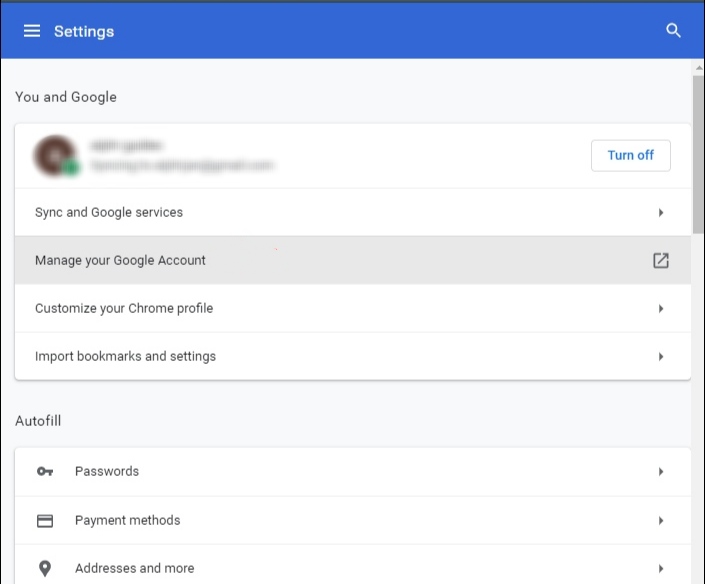In this screenshot of the settings for a Google account, the top portion features a prominent blue banner with the word "Settings" on the top left and a magnifying glass icon on the top right for search functionality. Directly beneath this banner is the section title "You and Google," followed by a blurred-out area likely representing the current user's account information, accompanied by a "Turn off" button on the far right.

Below this, a navigation panel presents several tabs for managing various aspects of the Google account. The tabs include "Sync Google Services," "Manage Your Account" (which is currently highlighted in gray), "Customize Your Chrome Profile," and "Import Bookmarks and Settings."

Further down, there is an "Autofill" section with options to manage "Passwords," "Payment Methods," and "Addresses and More." Each of these options is accompanied by specific icons: a key for "Passwords," a credit card for "Payment Methods," and a pin for "Addresses and More."

This comprehensive layout allows users to easily navigate and manage their Google account settings and Chrome preferences.